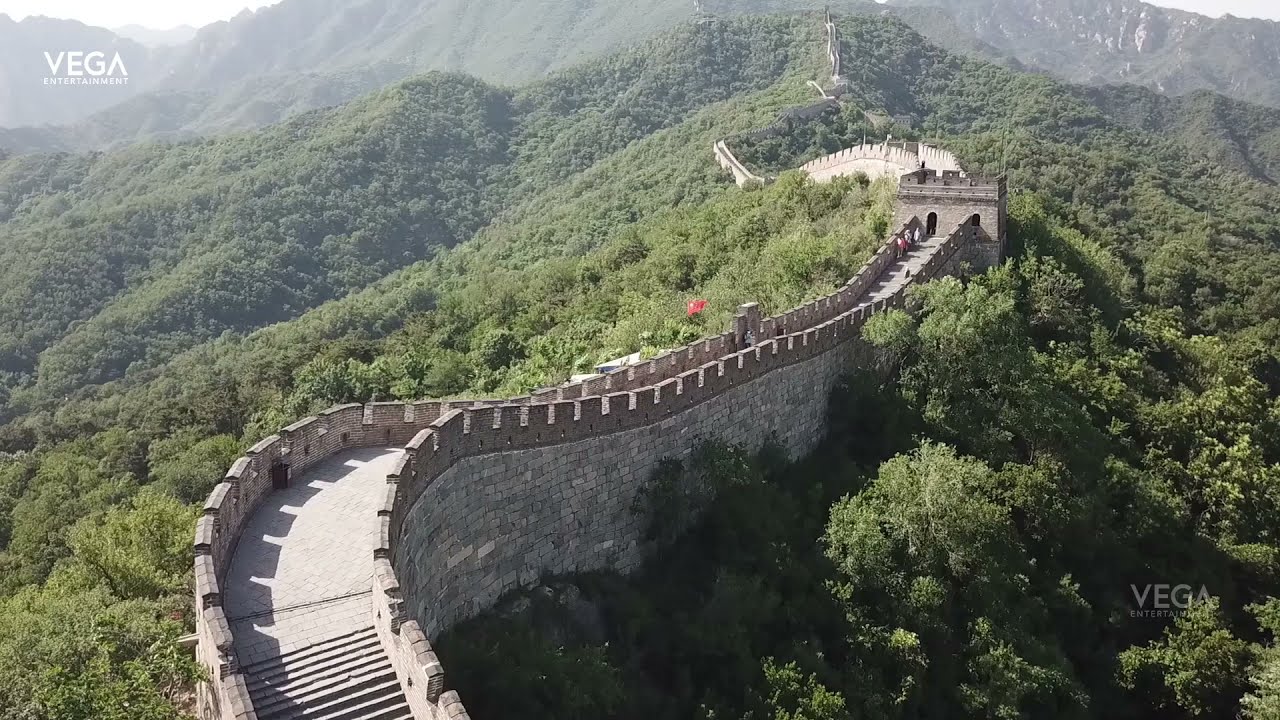This detailed aerial photograph depicts a winding section of the Great Wall of China, set against the backdrop of lush, verdant hills and forested mountain ridges. The wall, primarily constructed from a mix of gray, beige, and light brown stones, stretches diagonally from the bottom left to the upper right of the image, gradually fading into the hazy distance. Closer to the foreground, the structure's intricate dental molding and stone steps are clearly visible, emphasizing the wall's robust construction. Near the center of the photo, a small four-sided tower, possibly a historical lookout or rest stop, punctuates the continuous flow of the wall. Around this central point, a few tiny, human figures stand out against the grand scale of the structure, highlighting its immense size.

Flanking the wall on both sides, dense greenery composed mostly of tall trees adds a vivid touch of nature. Despite the overall clarity of the day, a light mist softens the distant mountain tops, suggesting a slightly hazy, sunny day. Notably, there is a small, red object—perhaps a flower or a flag—atop the wall, further adding to the visual interest. In the upper left and lower right corners, the text 'VEGA Entertainment' is prominently displayed in white capital letters, anchoring the image as a media or promotional piece.